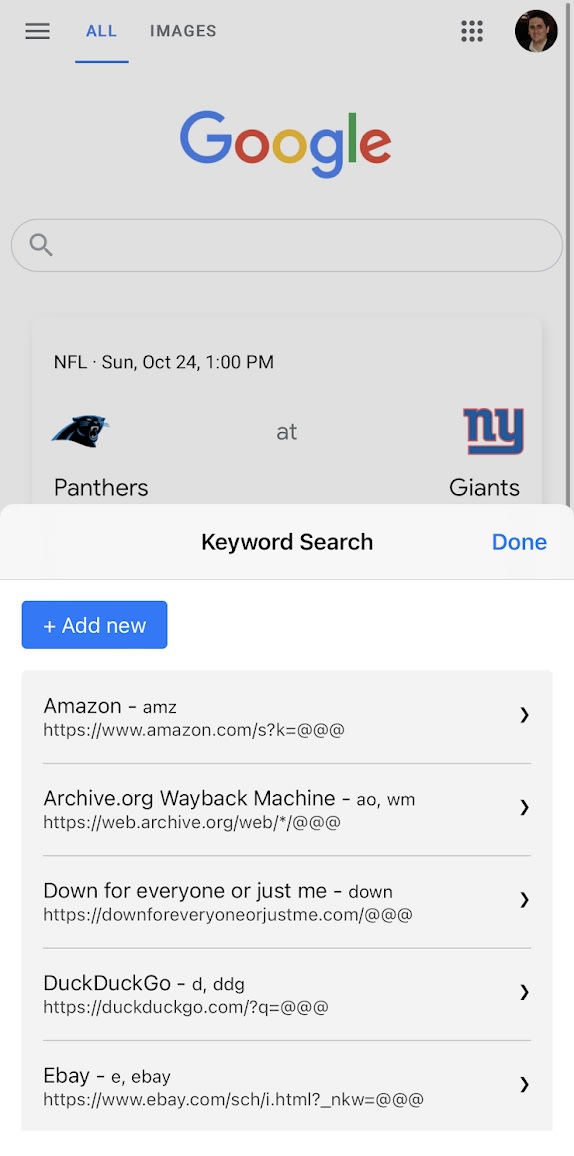A screenshot of a mobile website displays a Google search page. At the top left, options for "All" and "Images" are available, while a menu icon resides in the top right beside a profile picture. The Google logo is prominently centered at the top, followed by a search bar. Beneath the search bar are current NFL scores for Sunday, October 24th at 1 p.m. 

Superimposed on this backdrop is a white pop-up menu, emerging from the bottom of the screen, titled "Keyword Search." A "Done" button is situated at the top right of this pop-up. Below the "Keyword Search" title is a blue "Add New" button. To the left and underneath this button is a list of five website options: amazon.com, archive.org (Wayback Machine), Down for Everyone or Just Me, DuckDuckGo, and eBay. Each listing includes the URL below it and a small arrow on the right, suggesting additional actions or options.

The underlying Google page is slightly grayed out, ensuring the pop-up menu stands out. The purpose and function of the pop-up menu remain somewhat ambiguous based on the visual context provided.